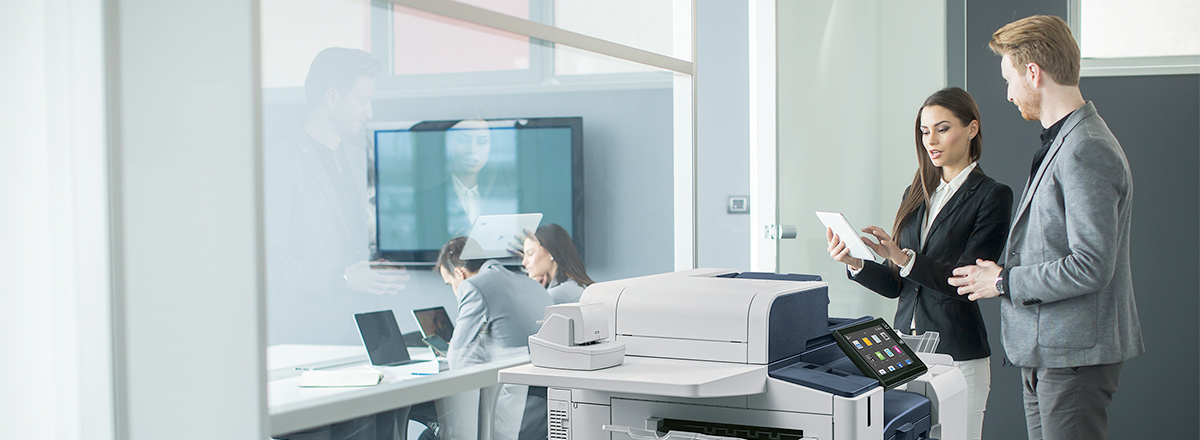In this image depicting a busy workplace setting, two individuals dressed in business attire are standing beside a sophisticated-looking copy machine with a large digital touchscreen. The woman, with brown hair and light-colored skin, is wearing a dark blazer, white button-up shirt, and white pants or skirt. She holds what appears to be a piece of paper or an iPad, concentrating on her task. The man next to her, also light-skinned with brown hair, is dressed in a gray jacket, black collared shirt, and gray pants, and he is looking at the item she is holding. Beyond them, through a clear glass window, there is a glimpse into a conference room, where two more individuals, presumably a man and a woman, sit at a white desk with gray walls. They are dressed in gray suits and absorbed in their laptops. On the wall of the conference room is a large-screen TV displaying a person speaking. This image captures the essence of a modern office environment, blending technology and professional interaction.